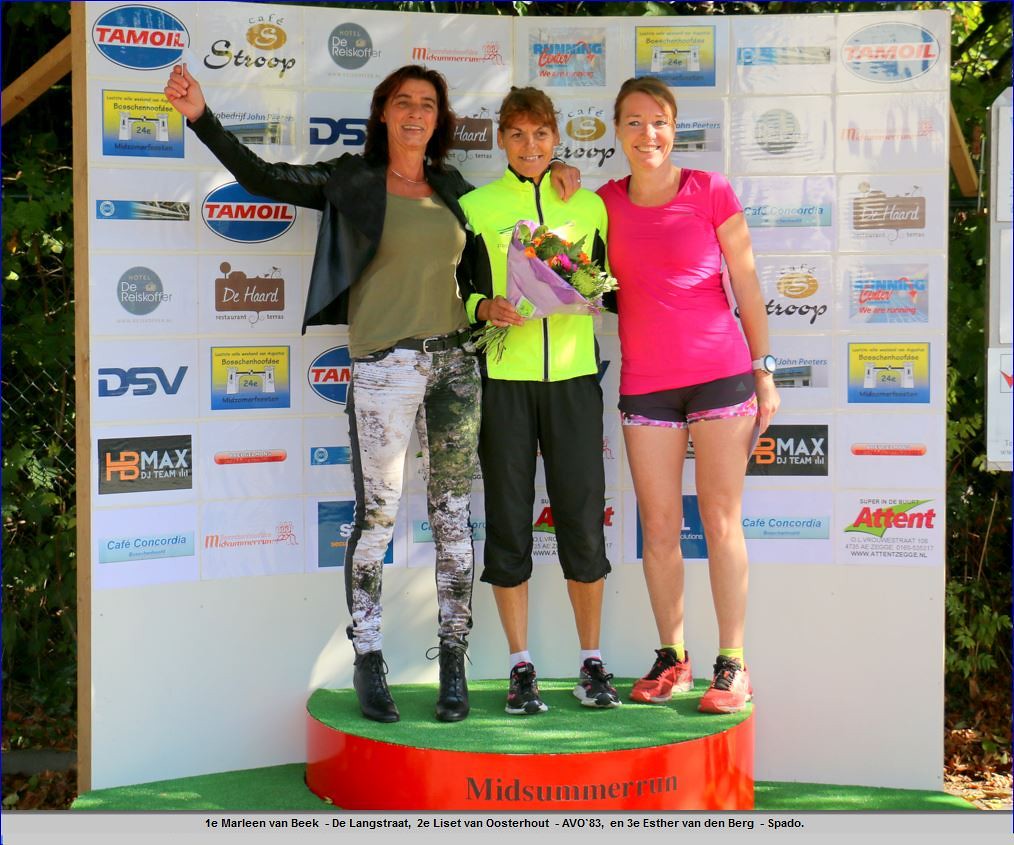Three women stand on a red and green platform that reads "Midsummer Run" in bold letters. They appear to have just completed a race. The woman on the right, wearing a pink short-sleeve t-shirt and small black shorts, glances towards someone off-camera, a white watch with a white face on her left wrist. In the middle stands a woman dressed in a neon green top with black accents and black pants, holding a bouquet of flowers. The woman on the left raises her right arm, clasping something unseen, and wears a black leather jacket over a green top, with multicolored white and green pants and black shoes. Behind them is a backdrop featuring evenly spaced, multicolored sponsorship logos, including Attempt, DSV, HB Max, and Dr. Hurd. A metal fence and trees are visible in the background, adding depth to the scene.